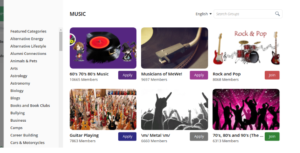This image appears to capture a section of a musical website, though its details are somewhat difficult to discern due to its small size. On the left side, there's a dark, grayish border which might be part of another image. This border darkens towards the top and features a couple of lines in the middle.

Adjacent to the border, there is a vertical, rectangular box containing various lines of text or information, though the small size of the image makes it unreadable. A scroll bar is visible next to this rectangular box, indicating that there might be more content below.

The main body of the website is centered around music-related content. The headline is written in bold, all-caps, black font. Beneath this headline, there are six media thumbnails.

The first thumbnail depicts a record player, showing the record itself with a purple button beneath it. The second thumbnail resembles the needle on a record, which also has a light purple button underneath. Further along, there is an image of a band featuring two rock guitars and a drum kit, with additional people visible in the bottom area of the image. Each thumbnail includes clickable buttons in blue, gray, and green positioned at the bottom, adding an interactive element to these media images.